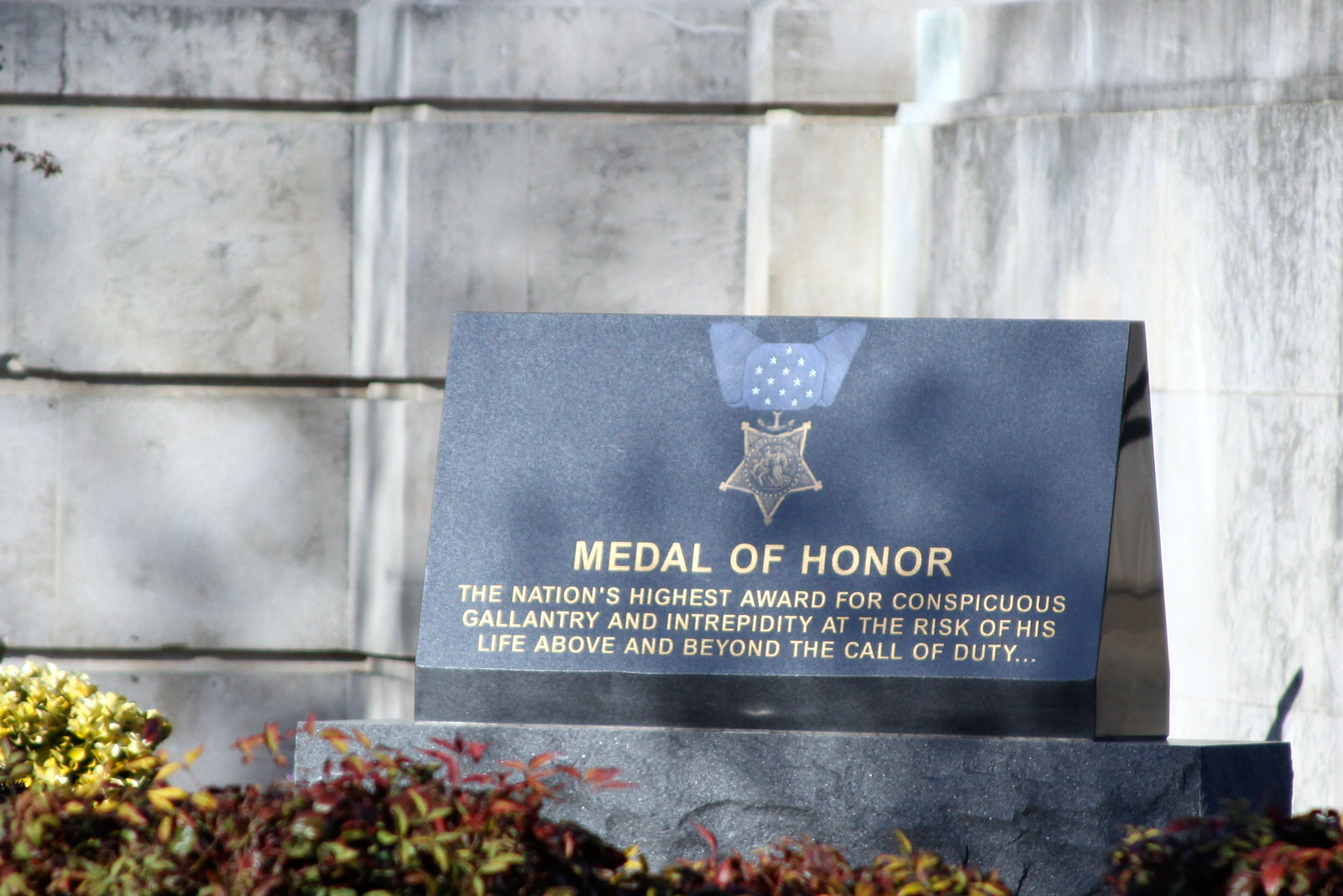This photograph showcases a solemn memorial stone that closely resembles a gravestone. The stone is crafted from dark granite, and the side visible in the image is inscribed with the words "Medal of Honor" in gold lettering. Beneath this title, the inscription reads, "The nation's highest award for conspicuous gallantry and intrepidity at the risk of his life above and beyond the call of duty." Above the text, a depiction of the Medal of Honor is prominently displayed, featuring a blue ribbon adorned with small white stars and a five-pointed gold star illustrating two soldiers. The memorial is set against a backdrop of a stone wall composed of gray and rusty silver-colored blocks, suggesting it is located in an outdoor setting, perhaps within a cemetery or memorial site. Surrounding the base of the stone is a variety of small ground cover vegetation in shades of green, yellow, and red.